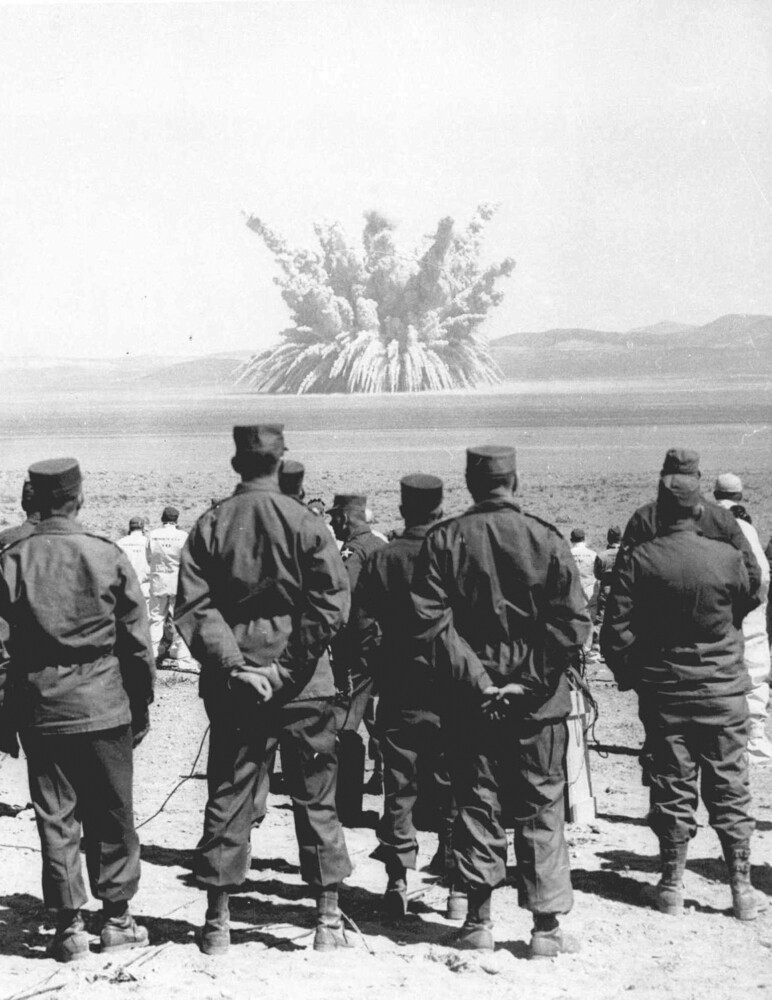This tall, black and white vintage photograph captures a group of soldiers and civilians witnessing a distant explosion. The image transitions from light gray at the top to a landscape featuring mountains and a barren, sandy area. 

In the foreground, several soldiers stand with their backs to the camera, clad in dark gray military uniforms and flat, circular hats. Some of them have their hands clasped behind their backs. Ahead of these soldiers, rows of individuals dressed in white uniforms without hats are also facing the explosion. 

The explosion itself, reminiscent of an eruption or firework, sends billowing streams of smoke and debris high into the air. The scene unfolds in what appears to be a desert or beach-like area, with the soldiers and civilians maintaining a calm demeanor as they observe the spectacle from a safe distance. The photograph's aged appearance evokes a time from "back in the day," though the exact era is unclear.